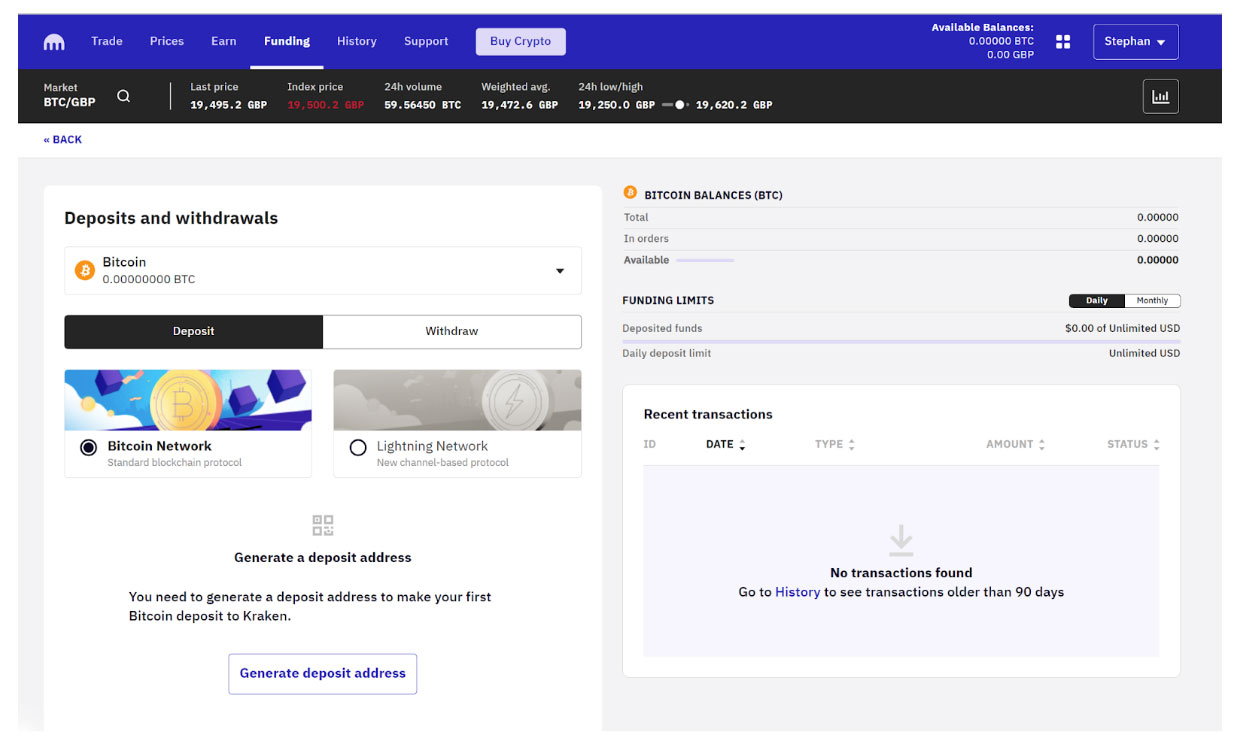This image showcases Steven's Bitcoin wallet on a cryptocurrency trading platform, specifically Kraken. At the top right corner, "Steven" is displayed with a downward-pointing white arrow, indicating a dropdown menu. The top section of the screen features a purple menu bar with a comb-shaped logo on the top left. The menu options, shown in white text, include "Trade," "Prices," "Earn," "Funding," "History," and "Support." The "Buy Crypto" button is highlighted prominently on the same menu bar. 

In the top right corner, the wallet's available balances are displayed as 0.0000 BTC and 0.00 GBP, with Steven's name beside them. Currently, the "Funding" tab is selected, indicated by a white underline beneath it and the label being in white, while the other menu options are in light gray.

Below the purple menu bar, a black line provides detailed market information, specifically the BTC/GBP pairing. It includes the last price, index price, 24-hour volume-weighted average, and the 24-hour low and high values of Bitcoin in pounds.

Further down, the interface splits into two sections against a white background. On the left side, the "Deposits and Withdrawals" section shows a zero balance for Bitcoin (0.0000 BTC). There are options to deposit funds via the Bitcoin network or the Lightning Network, along with options to withdraw funds or generate a deposit address. It instructs the user to generate a deposit address to make their first Bitcoin deposit, with a button provided to initiate this process.

On the right side, the Bitcoin balances are displayed, all showing zero, reiterating that no funds are currently held in the wallet.